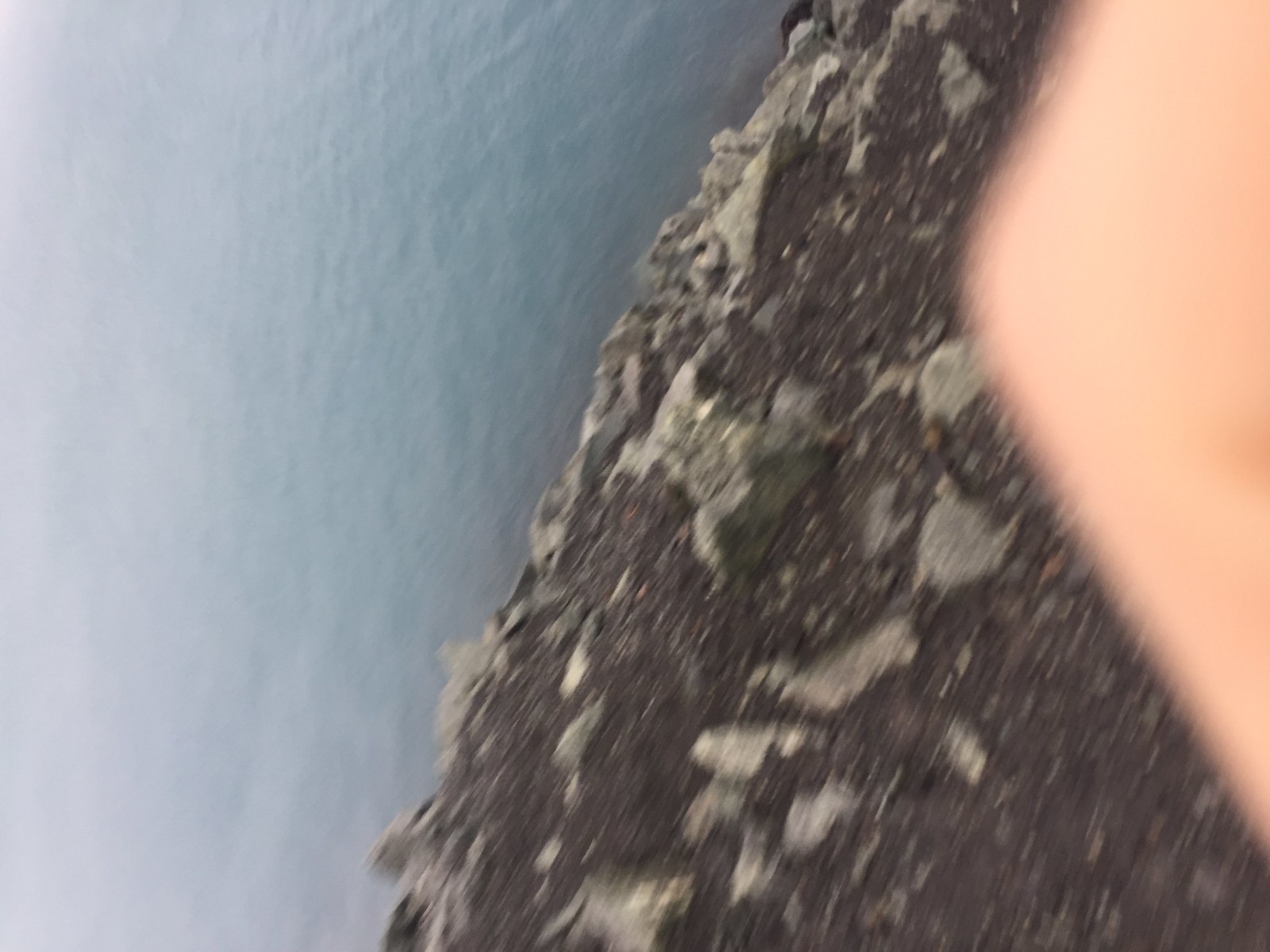A blurry image showing a rocky, brown dirt terrain meeting a body of water. The captured scene appears to be sideways, with the dirt and rocks on the right and the water on the left. The transition from land to water shows an increase in rock density as it approaches the water's edge, forming a rocky shoreline. The water is a vibrant blue, gradually fading into a lighter, whitish hue as it stretches out. Additionally, an indistinct object, possibly a finger, elbow, surfboard, or kayak, disrupts the scene, adding to the overall blurriness and making it challenging to identify specific details.